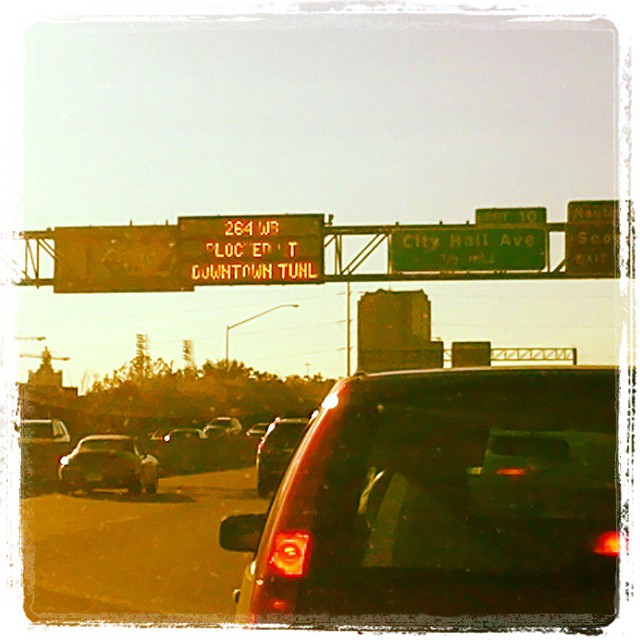In this image of a traffic scene, we observe a bustling highway environment from the perspective of a vehicle amidst congestion. Dominating the lower right corner is a nearby car, with its brake lights glowing. Visible details of this car include its rear window and a side window shaped like a short rectangle. To the left, additional vehicles populate the lanes; a car is positioned slightly ahead in the center lane, and another occupies the left lane.

A median wall separates the traffic moving in the opposite direction, where at least four cars can be discerned traveling toward us. Overhead, an assortment of road signs provides navigational information. A large sign prominently features the number "264" alongside the letters "WB" in red text. Although some letters are partially obscured or broken, "L-O-C-E-D" and the letter "T" are distinguishable. Below, the sign indicates directions to "Downtown" and "T-U-N-L" for tunnel. Next to it, a green city sign announces "City Hall Avenue," with an "Exit 10" designation enclosed in a rectangle above it. Partially visible, a brown sign shows some text, though the full content is obscured.

In the distance, tall telephone poles and light poles rise against the sky, emphasizing the urban setting of this busy interstate scene.